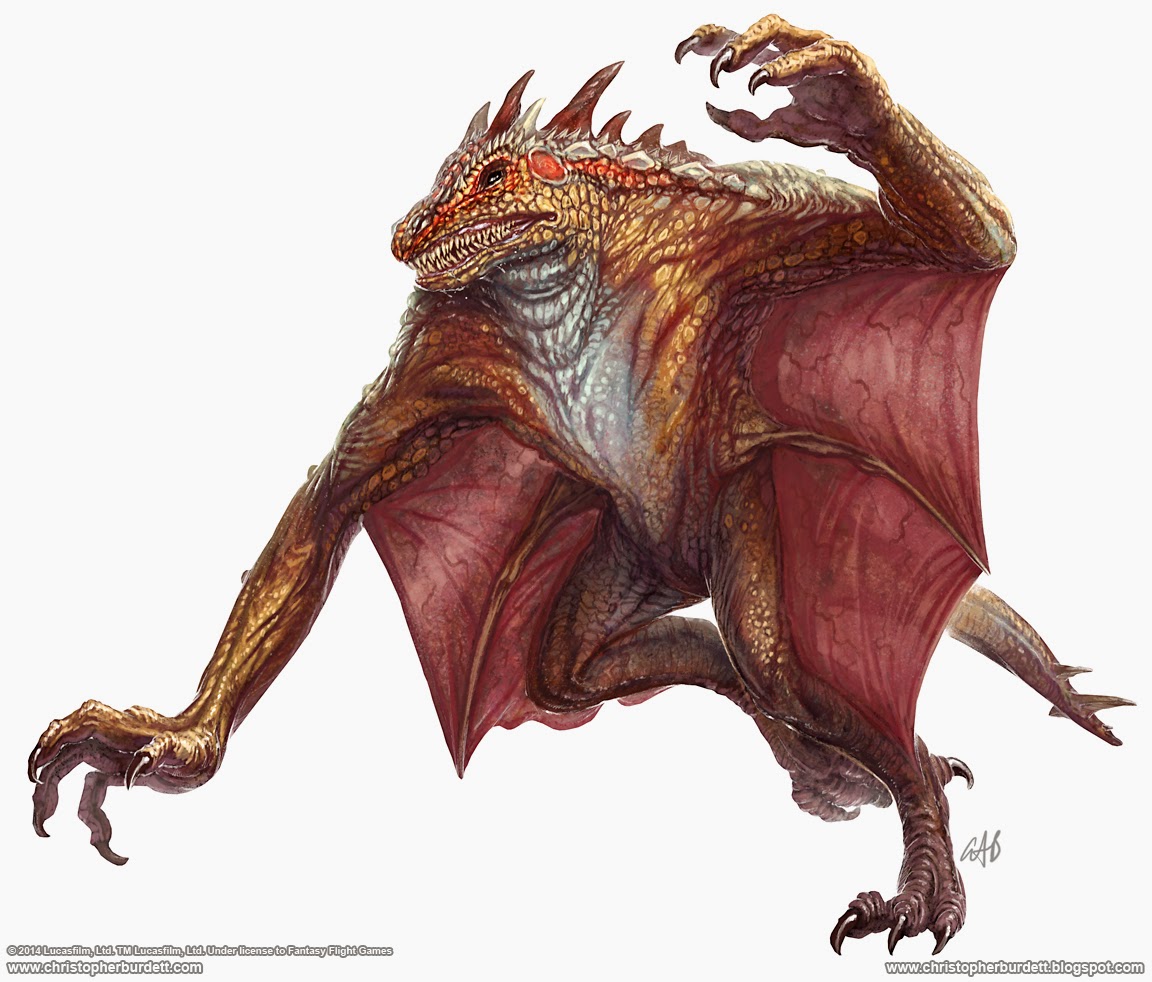This drawing depicts a mythological-looking creature set against a dull gray background, resembling a combination of an amphibian, bat, and lizard. The creature features an intricately detailed body primarily colored in yellow, orange, and deep red tones, with a distinct purple-red hue in certain areas, suggesting the presence of veins and arteries. It possesses bat-like wings with dark red webbing, well-defined long limbs ending in pointy black claws or talons, and large webbed feet similar to those of a bird. The creature's face resembles a hybrid of an alligator and a dinosaur, characterized by golden and orange hues, and is adorned with multiple spikes and ridges along the head and down the back.

The head has numerous sharp teeth visible in the open mouth, adding to its menacing appearance. Spikes on the tail and a muscular, stocky body enhance its otherworldly look. This fantastical beast features a scaly texture with a white underbelly and holds its left arm aloft, showcasing dark, elongated nails. The nape of its neck shades into gray, harmonizing with the overall color scheme. This illustration is from the website www.ChristopherBurdett.com and is copyrighted by Lucasfilm Ltd. in 2014 under a license to Fantasy Flight Games.